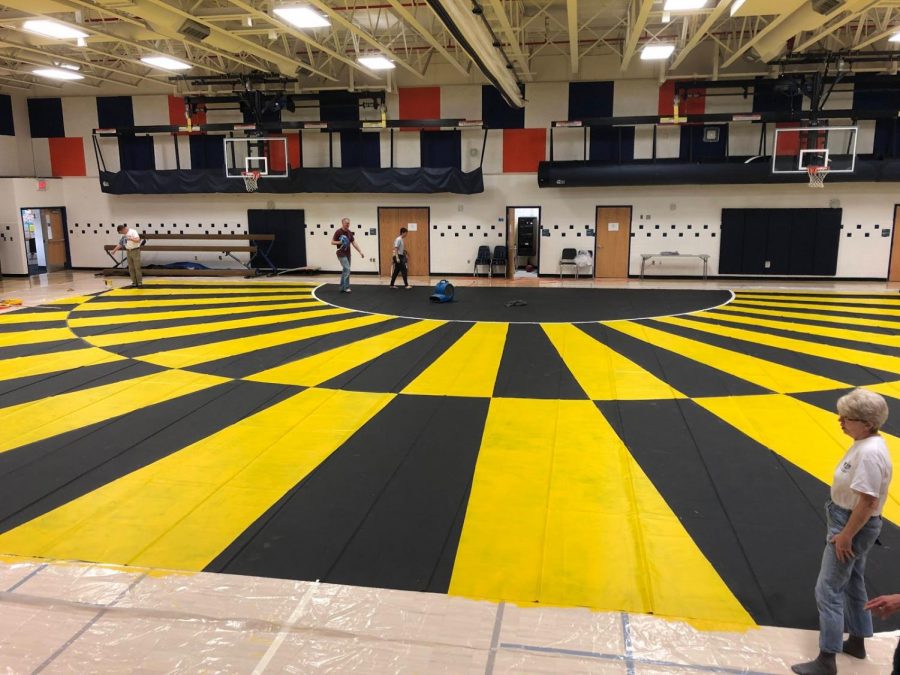This photograph captures the interior of a spacious gymnasium with distinctive design details and varied activities taking place. The gym floor is patterned in alternating sections of black and yellow with a prominent black semicircle outlined in white towards the front. An older lady, with gray hair, wearing a white t-shirt and blue jeans, stands in the foreground on a plastic tarp, seemingly involved in or observing the ongoing flooring work. To her left, a person's hand is visible, pointing towards something off-frame.

The background reveals a white wall adorned with a mix of navy blue, red, and orange squares, along with several beige and brown doors, two of which are open. Five doors line the wall, hinting at exits and other rooms. Several black chairs lean against this wall, contributing to the multi-functional aspect of the space. Two basketball hoops are mounted on the wall, underscoring the gym’s primary purpose as a sports facility.

Men, slightly out of focus, are seen near the back wall, possibly walking through the space or engaged in activities. Above, yellow beams and lights are visible, illuminating the entire area. The gym has a dynamic atmosphere, combining elements of construction and daily activity, reflective of a typical school or community center.